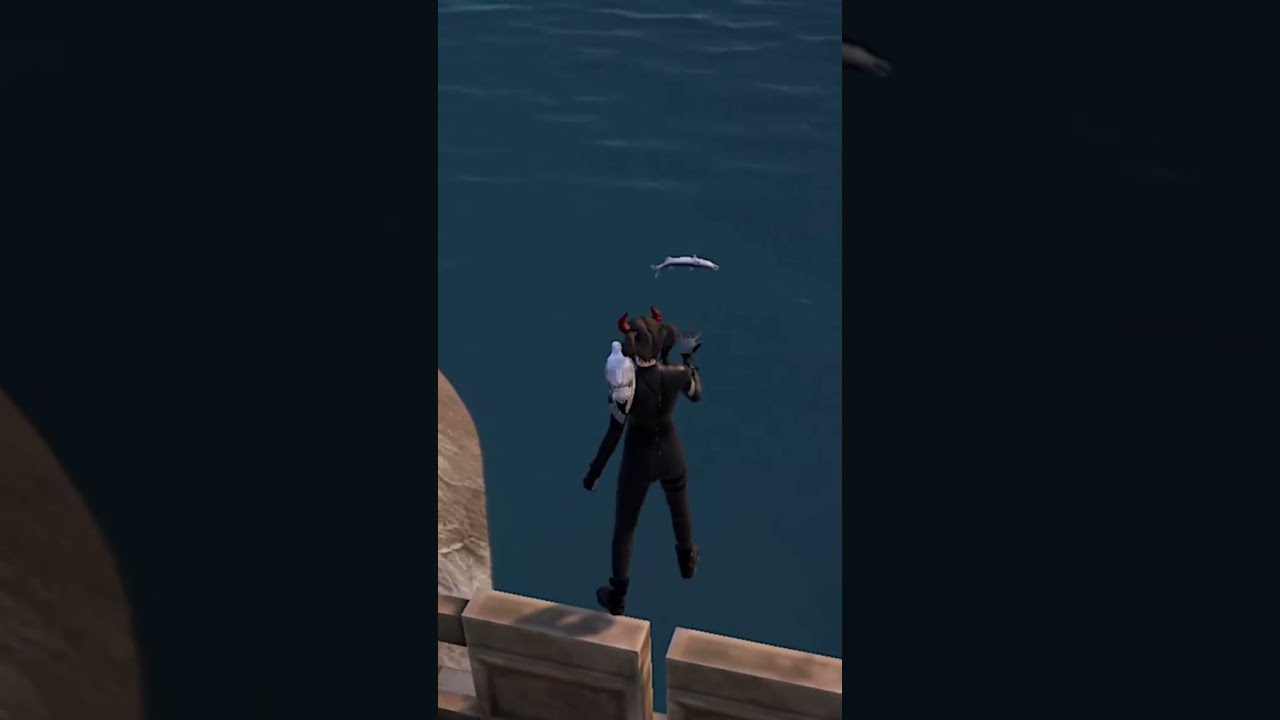A composite image showcases a woman with striking maroon devil horns protruding from either side of her head, her dark brown hair styled into ponytails. She's dressed in a black outfit and stands on the edge of a wooden boundary. On her left shoulder perches a light gray pigeon, while a dark black crow rests on her right shoulder. The background reveals a vast, blue sea, indicating her proximity to water. In one part of the triptych image, which appears to be a zoomed-in screenshot of an underwater game level, the woman dons a black scuba outfit, standing on underwater concrete blocks and facing a fish. Surrounding her are various aquatic elements, including a dead fish floating nearby. The central portion of the image displays the woman in another mystical scene, seemingly about to walk on the dark blue surface of water, ripples visible at the top of the image, with a fish swimming upside down towards her.